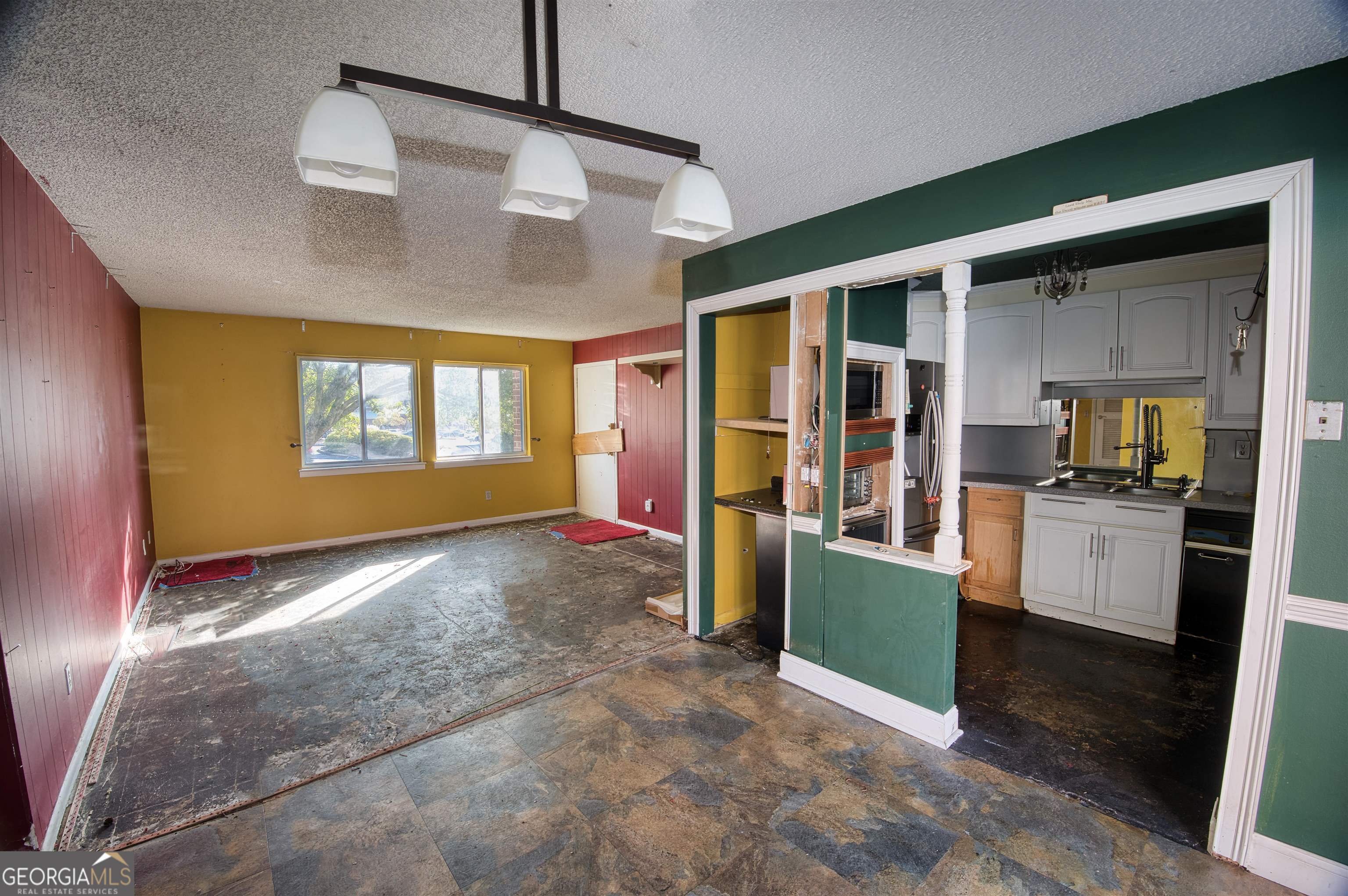This image depicts an unfurnished apartment, likely a real estate listing, showcasing a living room and kitchen viewed from the interior towards the front door. The kitchen, positioned on the right, is framed by green painted walls with white outlining on the door and some paneling. It features a fully stocked design with white shelves on top and bottom, accented by wood paneling. A black and silver oven and other electronics, possibly including a microwave, are integrated into the built-in shelves. Overhead, a central three-pronged light fixture with white bulbs and structures on a black pole illuminates the space. The living room boasts a variety of colorful paneling, with blue walls, red and yellow paneling on the front wall and doors. The floor, appearing to be an old marble with red pieces of carpet, suggests ongoing remodeling efforts. Windows are present on the yellow wall. The door at the entry has wood reinforcements. The diverse wall colors extend throughout the space and include red, yellow, white, gray, and more green. Light fixtures and a wooden platform adorn the ceiling, complementing the modern aesthetic of the kitchen. The image includes the text "Georgia MLS" at the bottom, indicating its listing source.